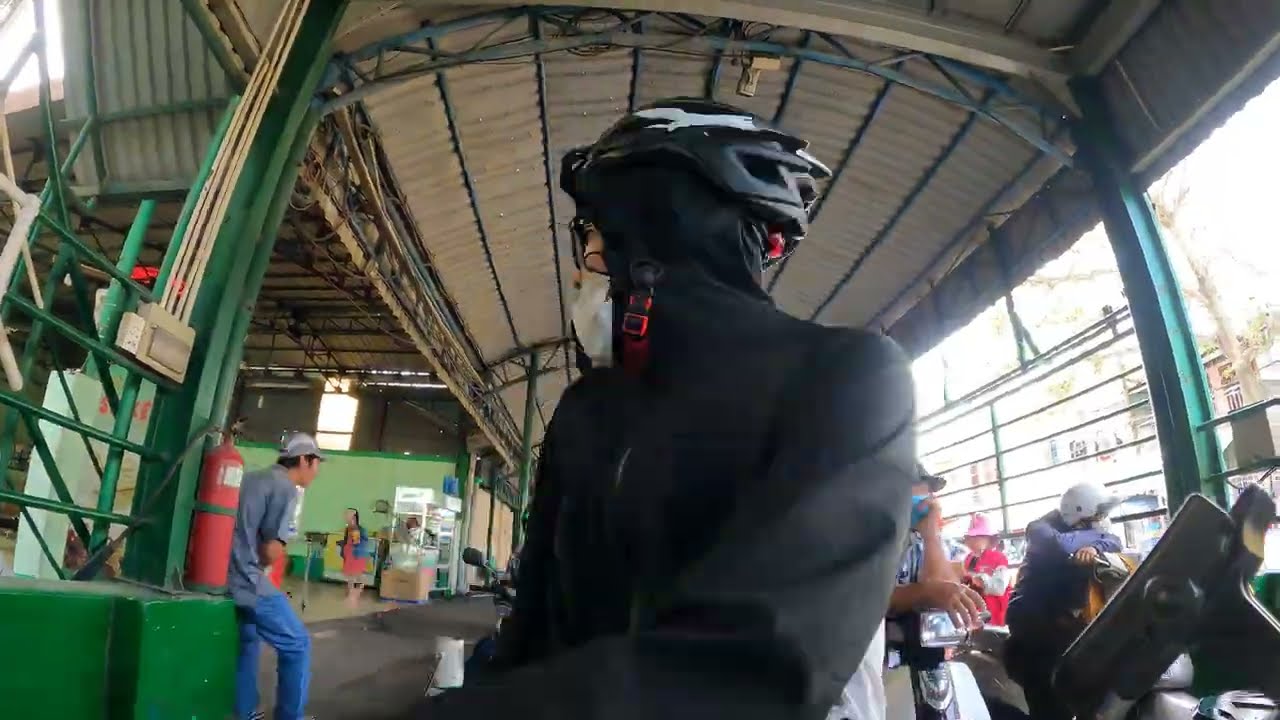In an outdoor enclosure with a gray metal roof, a man stands prominently in the center of the scene. He is wearing a black hoodie with the hood up and a black and white helmet over it. His face is partially obscured by glasses and a white mask. He is angled slightly to the side, with his head turned away from the viewer. Behind him, several people can be seen, some sitting on motor scooters as if waiting for something. To the left, a green post with green metal columns rises to the ceiling. Attached to the post is a red fire extinguisher, beside which a man in a gray shirt, blue jeans, and a hat is sitting with his back to us. Further back, a woman stands near what appears to be a kiosk or snack stand. The open area creates an impression of a platform, possibly a waiting area, with people sporadically looking out from underneath the roof.